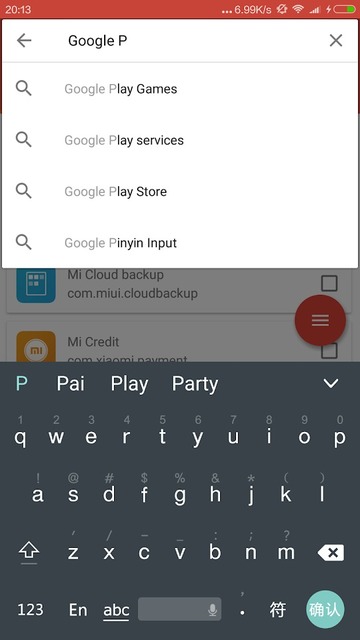A detailed screenshot captured on an Android phone shows the user actively engaging with an app. In the top right corner of the screen, a red banner displays critical phone features, including the time, which reads 20:13. Accompanying this are icons indicating battery life, data signal strength, Wi-Fi connectivity, an alarm muted indicator, and a notation of 6.99K-S.

The main focus of the image is the active search bar within the app interface, stark white against the screen, displaying the partial query "Google P" that the user is typing. Adjacent to this input field is a small gray 'X' for clearing the text and a leftward-pointing arrow on the left side for navigation.

Below the search bar, the familiar dark gray Android keyboard is visible, populated with predictive text suggestions like “P,” “pay,” “play,” and “party” in response to the user's input. The background of the app page, visible through a slight blur, features a red circle containing a three-line menu (commonly referred to as a hamburger menu) and two prominent clickable options named "MI Cloud Backup" and "MI Credit." The overall context suggests the user is searching for something related to Google within an app, possibly integrating or managing features and data on their Android device.